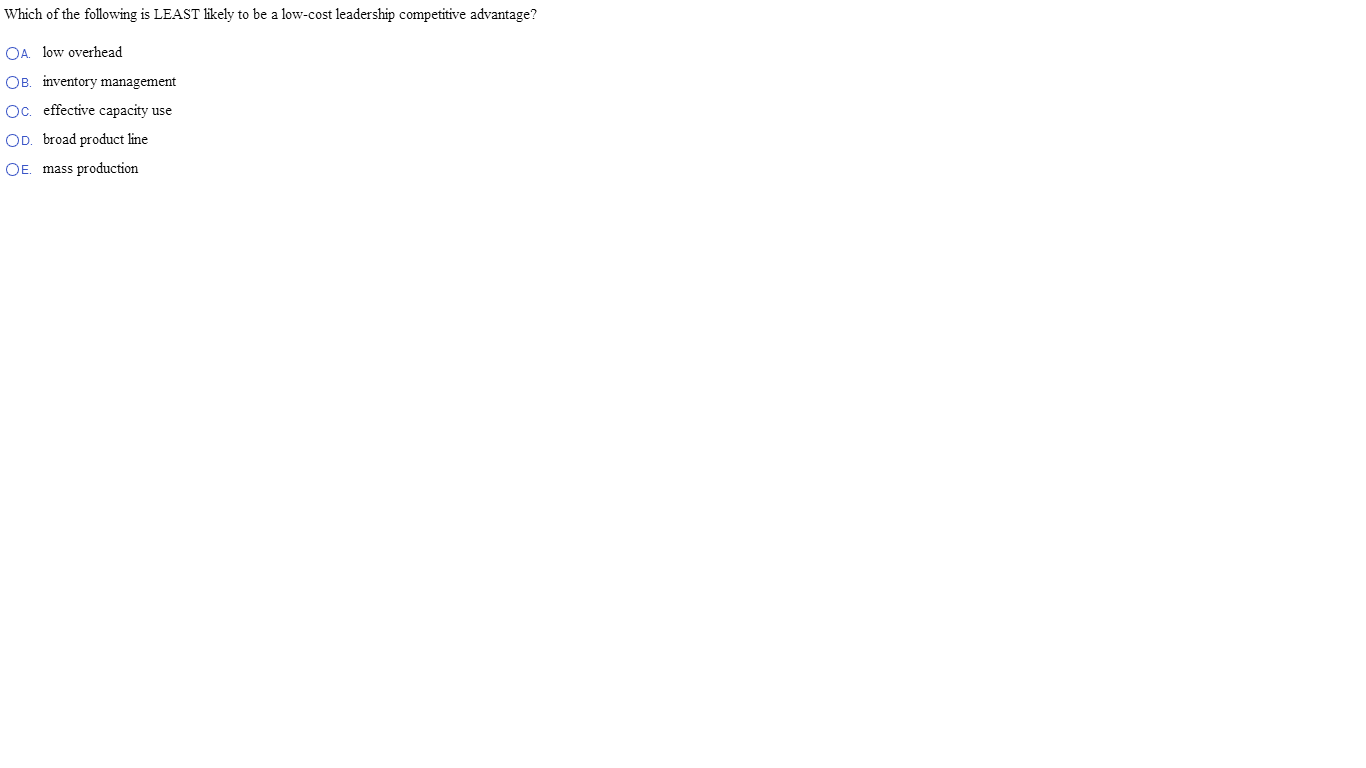The screen displays a quiz question centered in small print. The question reads, “Which of the following is LEAST likely to be a low-cost leadership competitive advantage?” The word “LEAST” is emphasized in uppercase letters. Beneath the question are five radio buttons labeled A through E, with none selected. The answer choices are as follows:

- A: low overhead
- B: inventory management
- C: effective capacity use
- D: product line
- E: mass production

Since the options use radio buttons, only one answer can be selected at a time, indicating that it is a single-choice question.